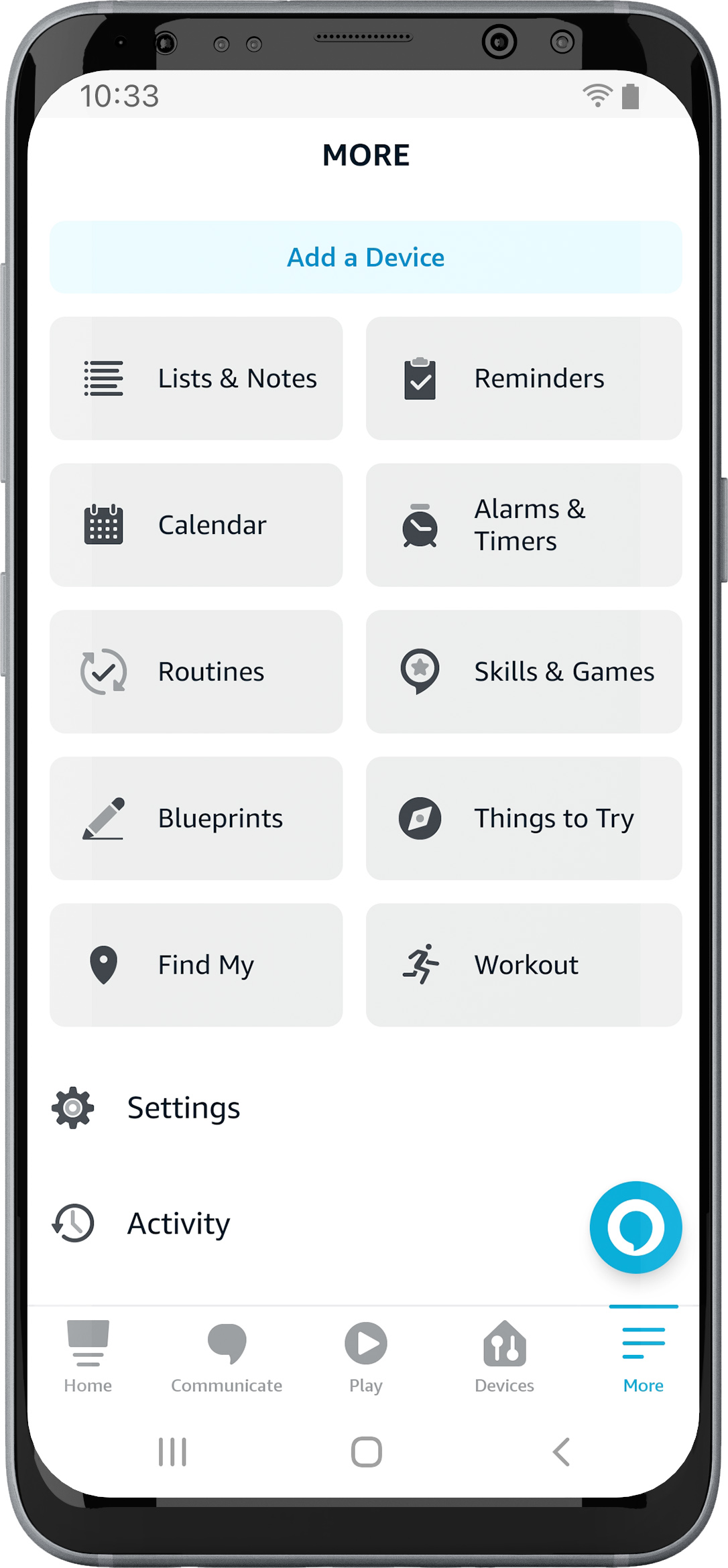The image displays a smartphone, reminiscent of an iPhone, with a sleek design featuring a black frame and black banners both at the top and bottom of the screen. At the top of the screen, against a white background, the time reads "10:33" in gray text. Nearby, icons for battery life and Wi-Fi signal are visible.

Centrally positioned on the screen is the word "MORE" in uppercase black letters. Beneath it, a banner in shades of blue catches the eye—powder blue transitioning to a darker hue in its center, which displays "ADD A DEVICE" with the letters A and D capitalized.

The lower part of the screen showcases a grid of light gray squares and rectangles with softened edges, organized into two distinct rows. The first row lists:
- LIST AND NOTES
- CALENDAR
- ROUTINES
- BLUEPRINTS
- FIND MY

The second row includes:
- REMINDERS
- ALARMS AND TIMERS
- SKILLS AND GAMES
- THINGS TO TRY
- WORKOUT

Additional options such as SETTINGS and ACTIVITY are also displayed on similar banners. A notable blue circle icon, resembling a small circle with a dot at the bottom, appears in this section, possibly indicating a voice assistant or notification.

Further down, the screen features a section with options labeled:
- HOME
- COMMUNICATE
- PLAY
- DEVICES

Lastly, a menu symbolized by three lines offers more choices, displaying options like MORE and BLUEPRINT.